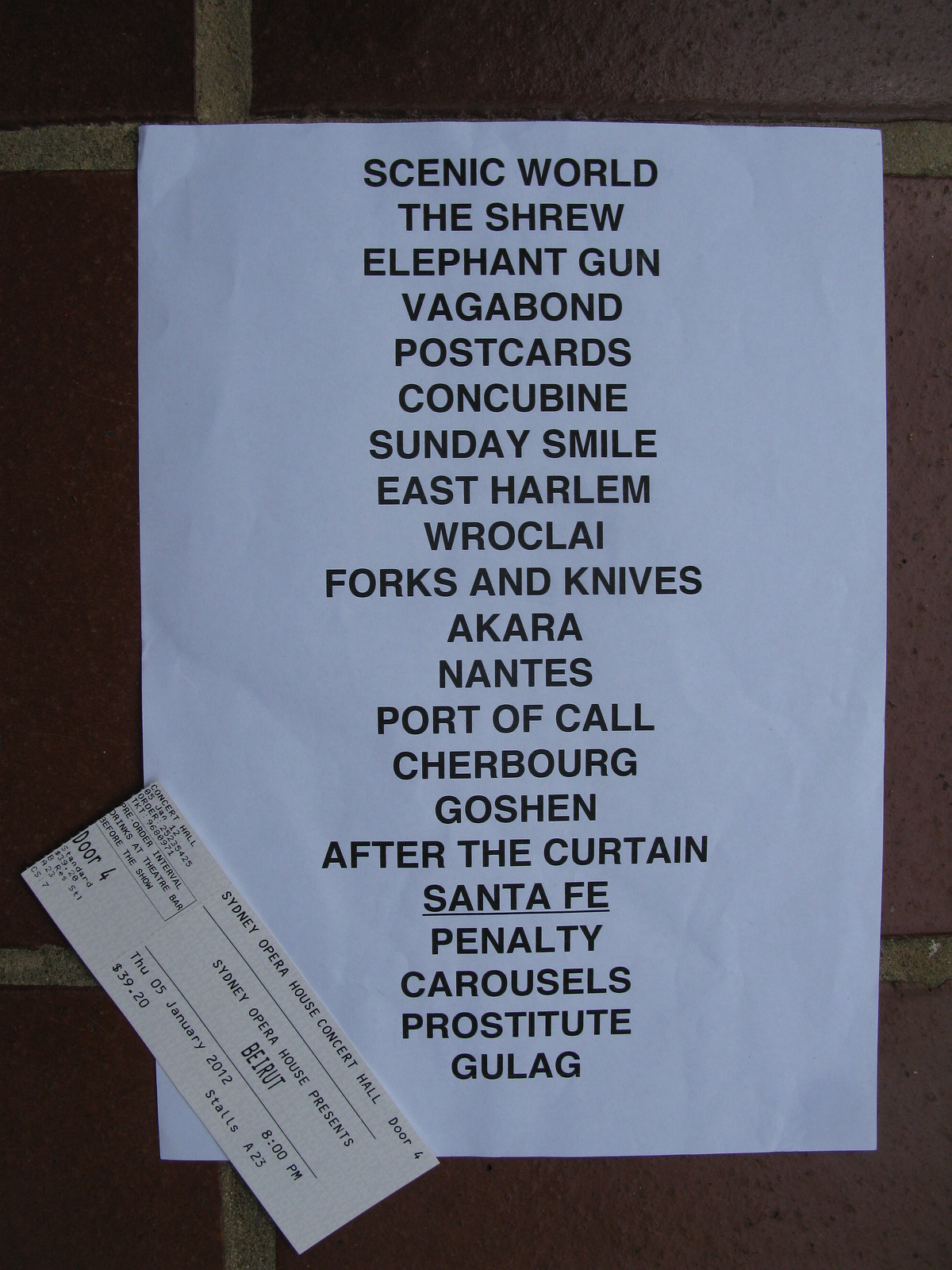This image depicts a white piece of paper adhered to the wall with block letters centered on the page, listing what appears to be a setlist of songs by the artist Beirut. The titles are as follows: "Scenic World," "The Shrew," "Elephant Gun," "Vagabond," "Postcards," "Concubine," "Sunday Smile," "East Harlem," "Roleclaw," "Forks and Knives," "Akira," "Nantes," "Port of Call," "Cherbourg," "Gauchin," "After the Curtain," "Santa Fe," "Penalty," "Carousels," "Prostitute," and "Gulag." In the lower left corner, a ticket stub is affixed to the paper at a downward right angle. This ticket stub indicates admission to a concert at the Sydney Opera House featuring Beirut, held on Thursday, January 5, 2012, with tickets priced at $59.